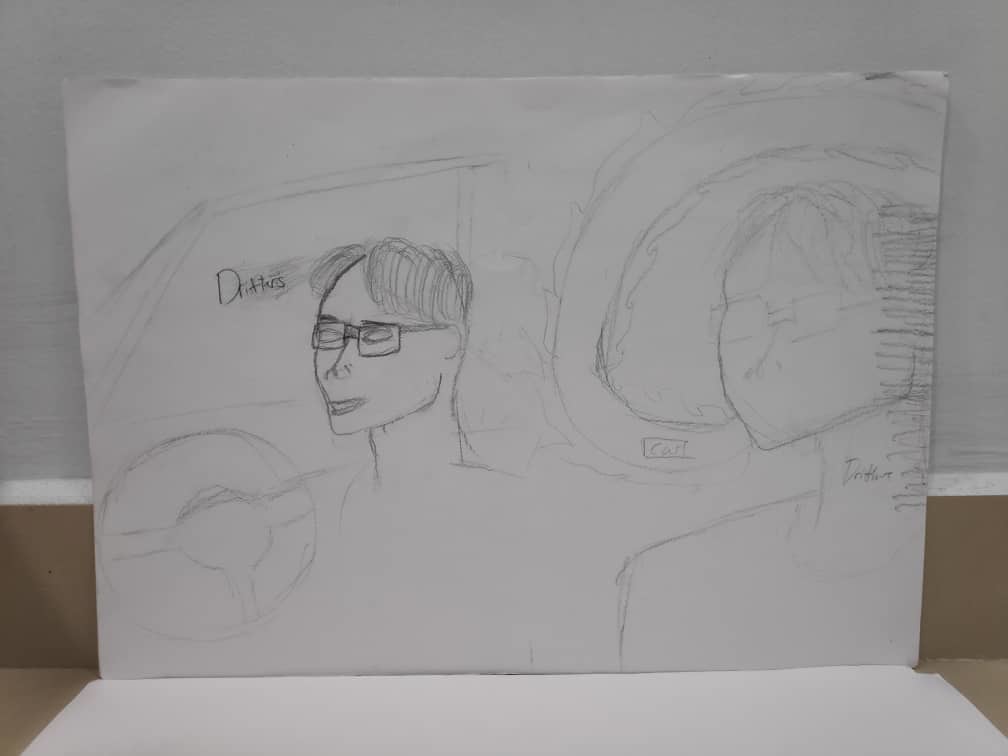The image is a highly detailed pencil drawing on a plain white sheet of paper, propped up against a white wall with a light brown baseboard and tabletop below it. The drawing depicts two similar-looking individuals possibly inside a car. The most prominent figure is on the left side, with long stringy hair parted in the middle, wearing rectangular black-rimmed glasses and a half-smile. This person is positioned behind what appears to be a steering wheel, though the car may be parked since their eyes are closed. Below their neck, barely legible text that seems to spell out "detective" or "doctor" can be seen.

To the right of the main figure is a lightly sketched, almost shadow-like version of the same or a similar person, though their features are rendered in fainter lines, suggesting either a preliminary sketch or a depiction of another individual sitting beside the first. In the background, there appears to be a swirling pattern along with what looks like a car window, reinforcing the vehicular setting. The word "drifters" is printed in the background, adding a narrative element. The level of detail in the faces, particularly the glasses, nose, mouth, and even the hint of an eyebrow, contrasts with the more suggestive rendering of the car and background elements.